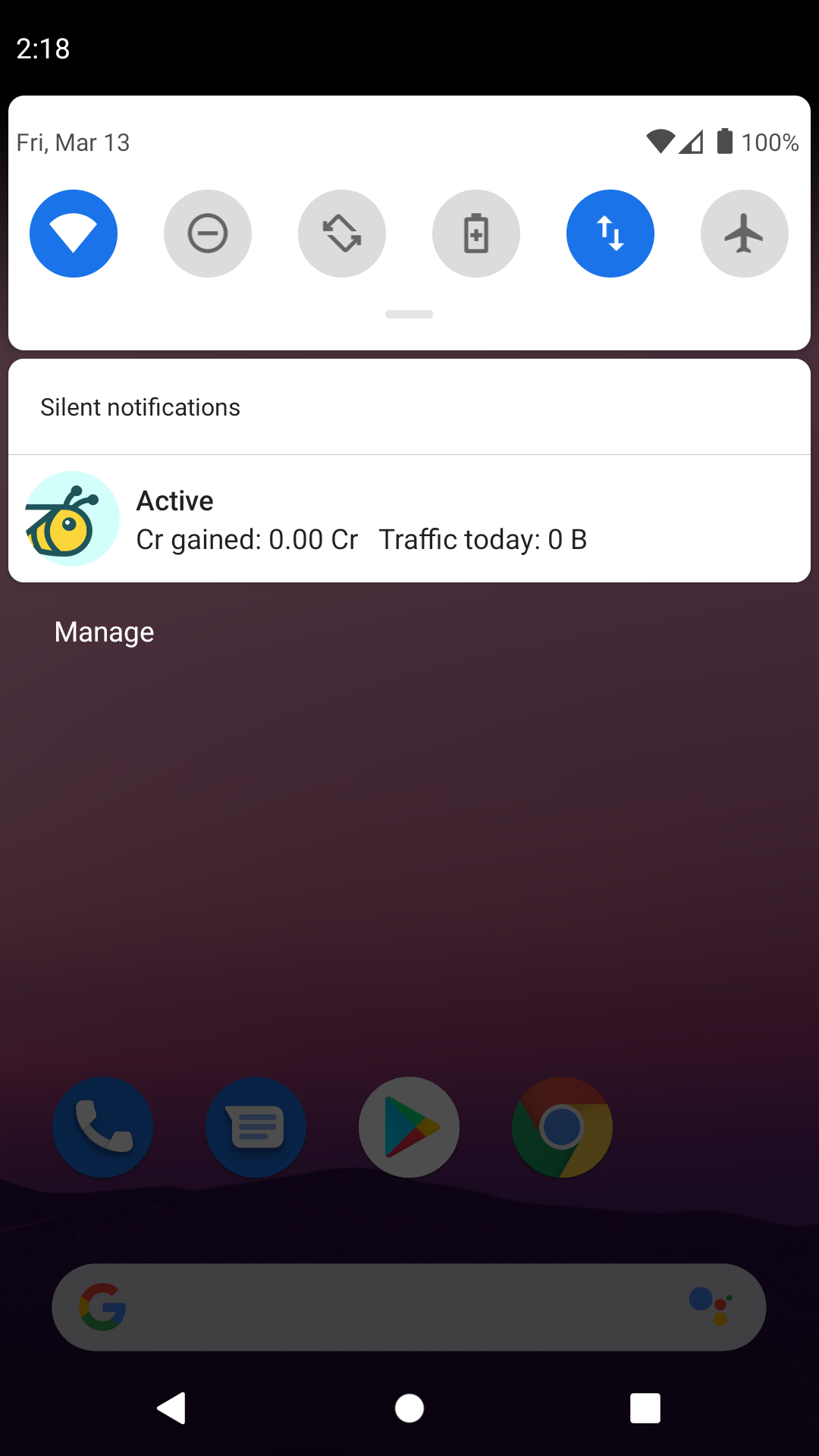This image is a screen capture of a cell phone displaying its swipable top-down menu on the home screen. In the upper left corner, in white text, it reads "2:18". Below, the drop-down menu of the Android operating system is shown with the heading "Friday, March 13th". The status bar indicates a battery level of 100%, partial cellular service, and full Wi-Fi connectivity.

There are six icons displayed in the quick settings panel. The Wi-Fi icon is blue, signifying it is active, while the following icons are grayed out, indicating they are inactive: Do Not Disturb, Screen Rotation, Battery Saver, and Airplane Mode. The blue up and down arrows represent mobile data, indicating its active status.

Beneath these icons, there is a section labeled "Silent Notifications," followed by a thin gray line. An app notification is present, characterized by an icon with a 'B' on a blue background. The notification text reads: "Active CR gained: 0.00 CR, Traffic today: 0B," with a "Manage" option below.

In the background, the phone's home screen is visible, featuring a purple mountain-themed wallpaper. The home screen also includes a Google search bar at the bottom and four app icons: Google Chrome, Google Play Store, the Messenger app, and the Phone app.